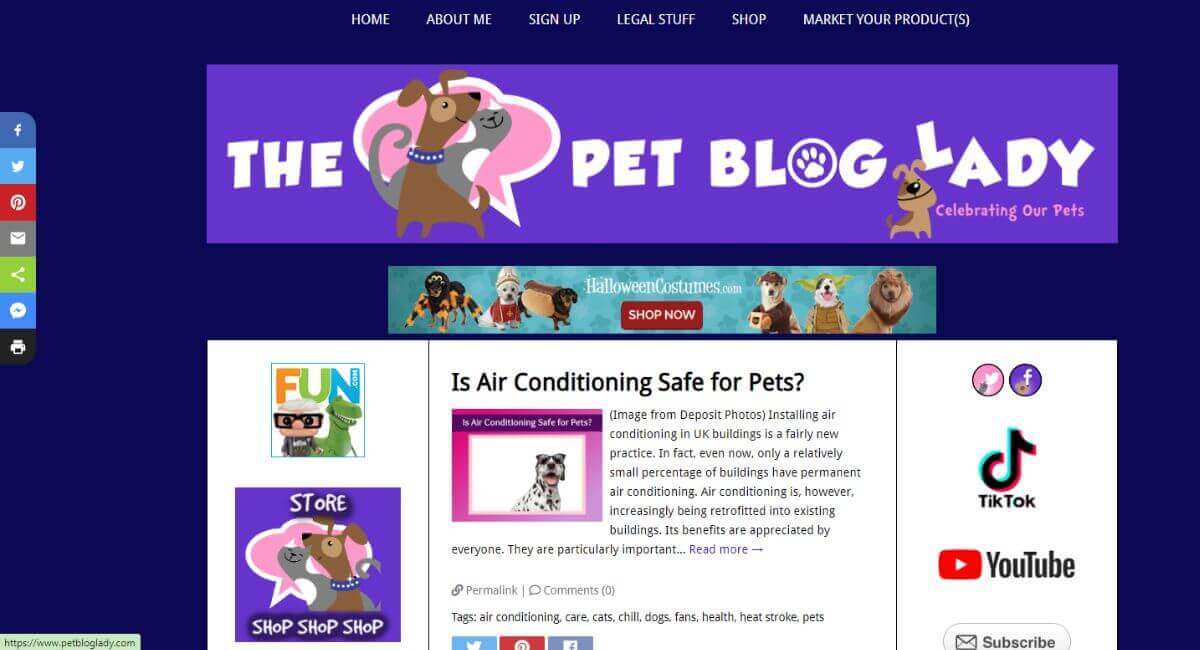In this image, we are viewing a web page prominently featuring a periwinkle banner at the top center. The banner displays the title "The Pet Blog Lady" in white block text. Accompanying the title is an illustration of a cartoon-like dog and cat standing in front of a pink cloud. In the lower right corner of the banner, there is a small dog with the phrase "celebrating our pets" written in fine print next to it. 

On the left side of the web page, there is a vertical array of colorful icons for various social media and sharing options, arranged from top to bottom as follows: Facebook, Twitter, Pinterest, email, share, and message. Beneath these icons is a white printer icon. Further down in the lower left corner, the website URL "https://www.petbloglady.com" is displayed. 

Below the banner, set against a white background, the blog post title reads: "Is air conditioning safe for pets?" To the right of this title, there's an introductory text that states: "Installing air conditioning in UK buildings is a fairly new practice."